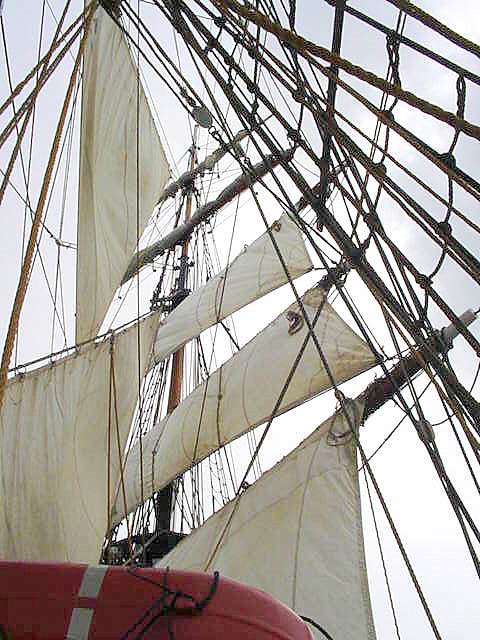This full-color photograph, taken on a mostly cloudy day with occasional glimpses of blue sky, captures the intricate details of a classic wooden sailing ship reminiscent of an old-style or pirate vessel. The image, shot from the deck looking upward, showcases an array of masts and a complex network of ropes, lines, pulleys, and supports stretching in every direction. Some of the masts feature partially opened off-white canvas sails, slightly worn from use, while others remain bare. The photograph includes approximately five sails, with larger sails positioned on the left side of the image. A red and gray-trimmed portion of the ship is visible at the bottom, alongside what appears to be a red life raft or life ring with white stripes. The cloudy sky serves as the backdrop, accentuating the grandeur and complexity of the ship's rigging and masts.